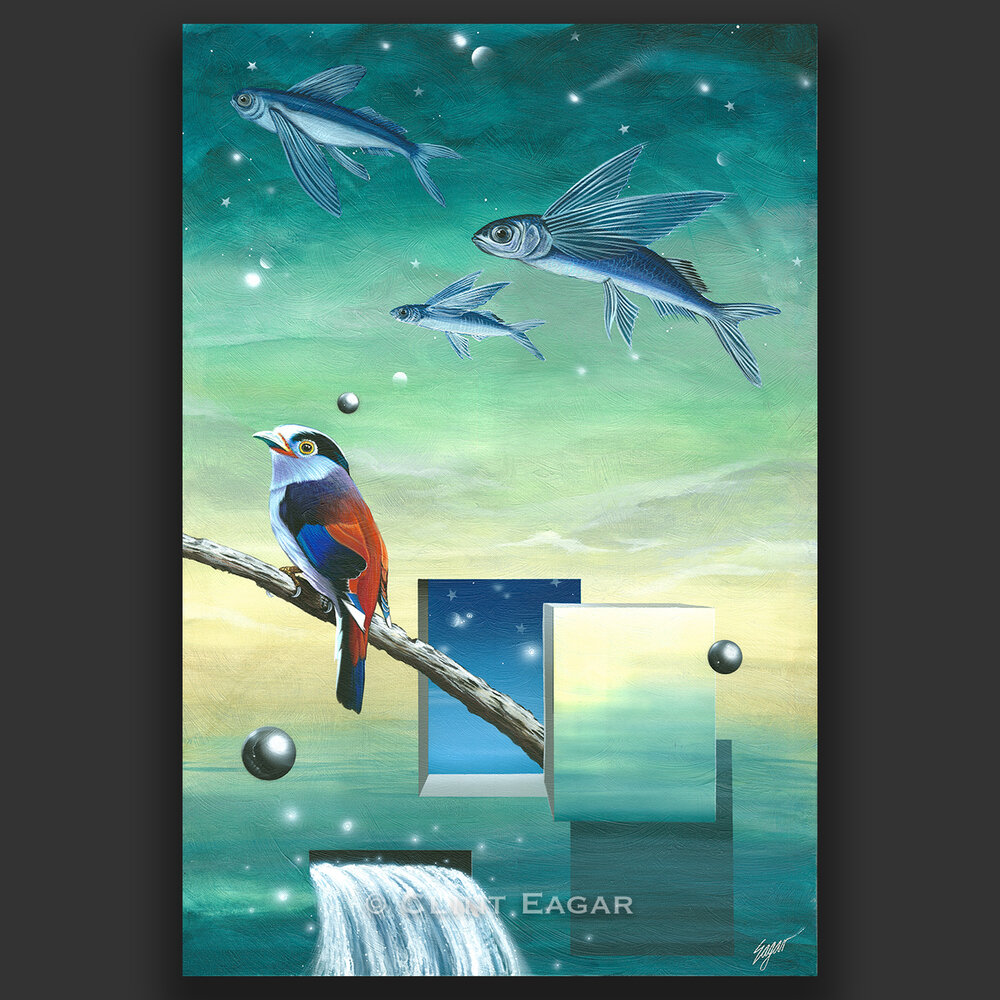The surreal artwork is a mesmerizing blend of water, fish, and sky. Central to the image is a vibrant bird perched on a wooden stick, which intriguingly pierces through a portal-like frame. The bird sportingly flaunts a striking mix of red, blue, and black plumage, an orange beak, yellow eyes, and a white underbelly, with flat feathers. Above, the night sky is dotted with stars and a moon, transitioning from dark at the top to a lighter blue at the horizon. Adding to the dreamlike quality, three flying fish with wings soar through the sky. The composition includes three floating metallic spheres, placed strategically around the bird. Below the bird, water flows through a cutout, and the painting is signed "Clint Eager" at the bottom. The colors are predominantly turquoise and blue, evoking an otherworldly, abstract atmosphere.